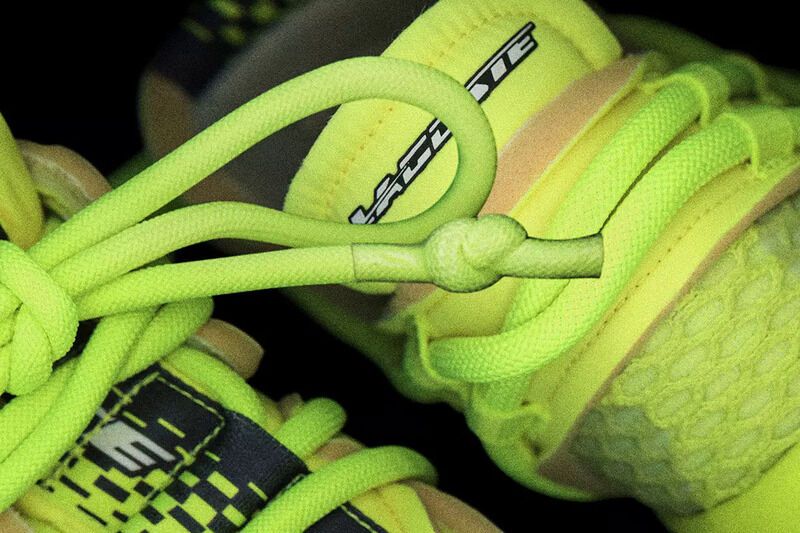This image presents a striking, extremely close-up photograph of a pair of athletic shoes, prominently showcasing the thick, fluorescent lime green laces intricately tied in knots and bows. The sneakers themselves feature a mix of tan or beige and black coloration, with a noticeable lime green mesh around the laces and possibly on the heel. The branding on one shoe vaguely reads "Lacoste" or something similar. The image is taken at an angle, tilting the shoes diagonally within the frame, and is set against a black background that emphasizes the vivid colors. The shoes appear almost abstract at first glance due to the extreme proximity of the shot, requiring a moment to discern their true nature. The interior of the shoe is gray, further adding to the color contrast.